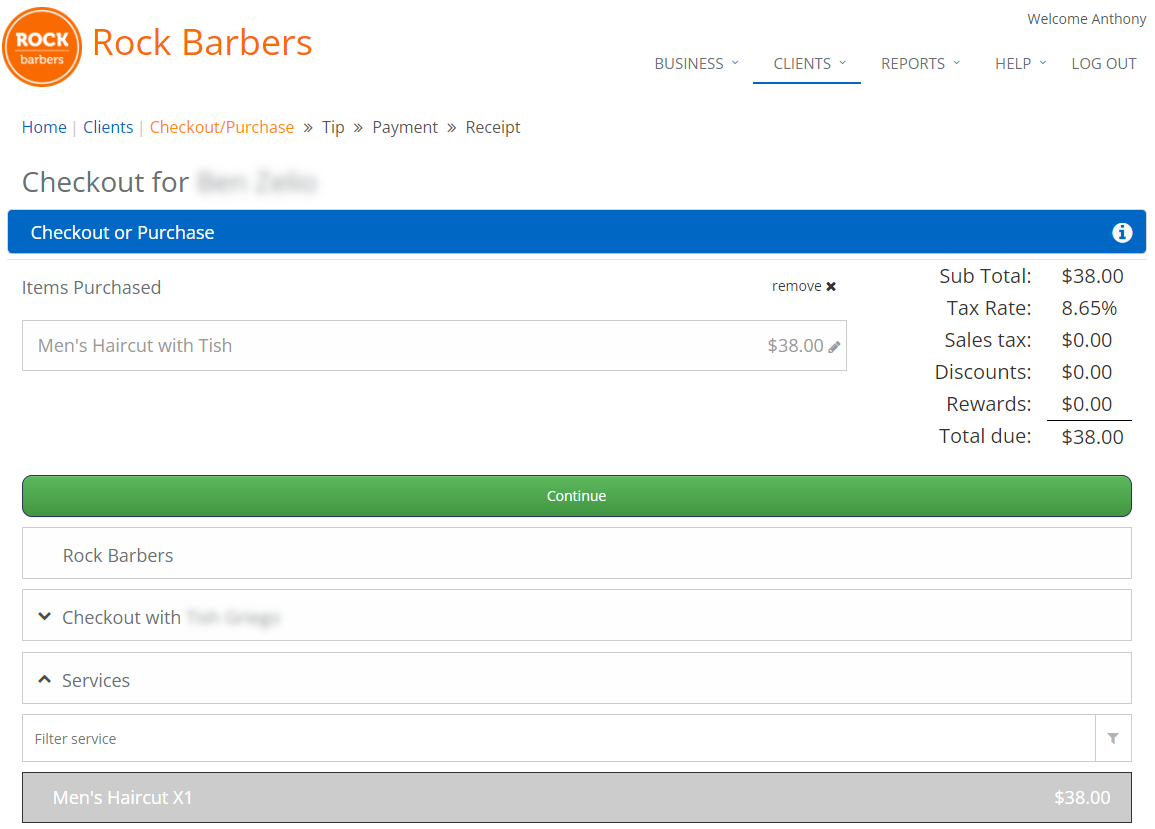At the top left corner of the interface, the word "Barbers" is displayed in bold, orange letters. On the top right corner, there is a menu with options that read: "Home," "Clients," "Checkout/Purchases," "Tip Payment," and "Receipt," listed in sequence. Another smaller text on this corner reads "Business," "Clients," "Reports," "Help," and "Logout." Beneath this, it warmly greets the user with "Welcome, Anthony."

A blue underline highlights the "Clients" menu option. The main content area shows a blurred checkout screen that primarily states "Checkout or Purchase Items." Below this heading, there's a list of items starting with "Men's Haircut with Tish - $38," followed by a detailed breakdown: 
- Subtotal: $38
- Tax Rate: 8.65%
- Sales Tax: $0.00
- Discounts: $0.00
- Rewards: $0.00
- Total Due: $38

A prominent green button with white text labeled "Continue" appears underneath the listed amounts. Following this button, the text "Rock Barbers" is displayed, alongside another "Checkout with" label, accompanied by a dropdown box that features a blurred-out name.

Further down, there's a "Services" section with a filter dropdown, currently set to "Men's Haircut x1 - $38."